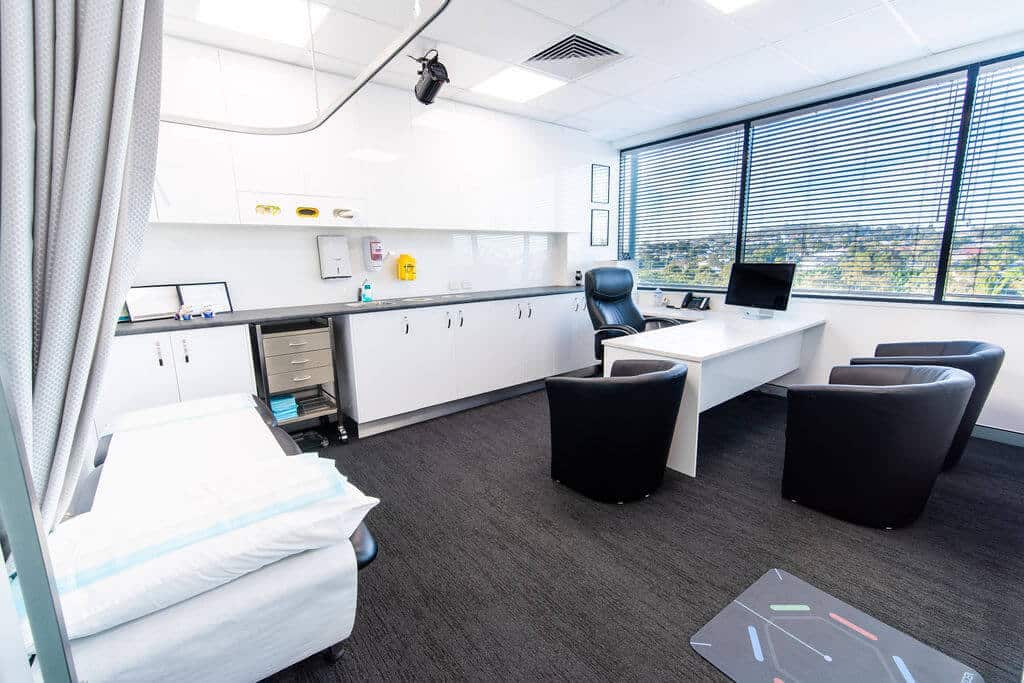This image depicts a sleek, contemporary doctor's office characterized by its clean, modern design. The space features stark white walls adorned with several cabinets and a sleek, stainless steel set of drawers on wheels, which likely serve as a mobile medical cart. A dark, expansive counter holds framed diplomas or certificates leaning against the wall. The office’s focal point is a large, well-appointed desk with a high-backed, leather office chair and a computer monitor positioned on top. Across from the desk, a set of modern, C-shaped leather chairs provide seating for consultations. To the left of the desk, a bed designed for patient examinations is covered with a white sheet and pillow, flanked by gray curtains for privacy. Above, ample lighting ensures a bright, clinical atmosphere. Just beyond the examination area are three large windows with partially open blinds, through which a distant view of greenery and perhaps other buildings can be seen. The room features dark flooring with a rubber mat near the examination bed, contributing to the overall sense of functionality and cleanliness.